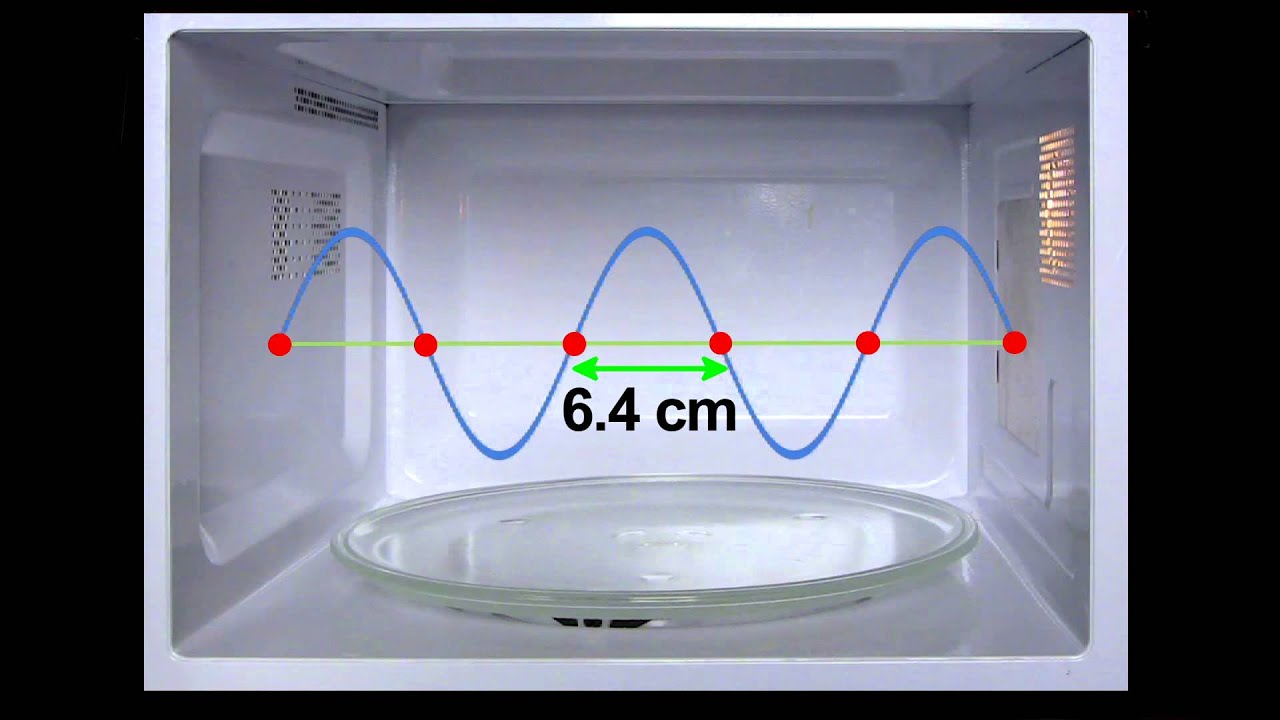The image depicts the interior of a white microwave oven with a clean, clear glass rotating plate at the bottom. The microwave door is not visible, and the unit is set against a black background, accentuating its clean, illuminated interior. A green light spans horizontally from the left to the right side of the compartment, intersected by six red dots. Connecting these dots is a blue sinusoidal wave, which underscores their alignment. Notably, the distance between the third and fourth dots is marked as 6.4 cm, with arrows pointing left and right to illustrate this measurement. The right side of the microwave emits an orange light, adding a dynamic visual element. This illustrative overlay and accompanying textual details emphasize the wavelength measurement within the microwave.